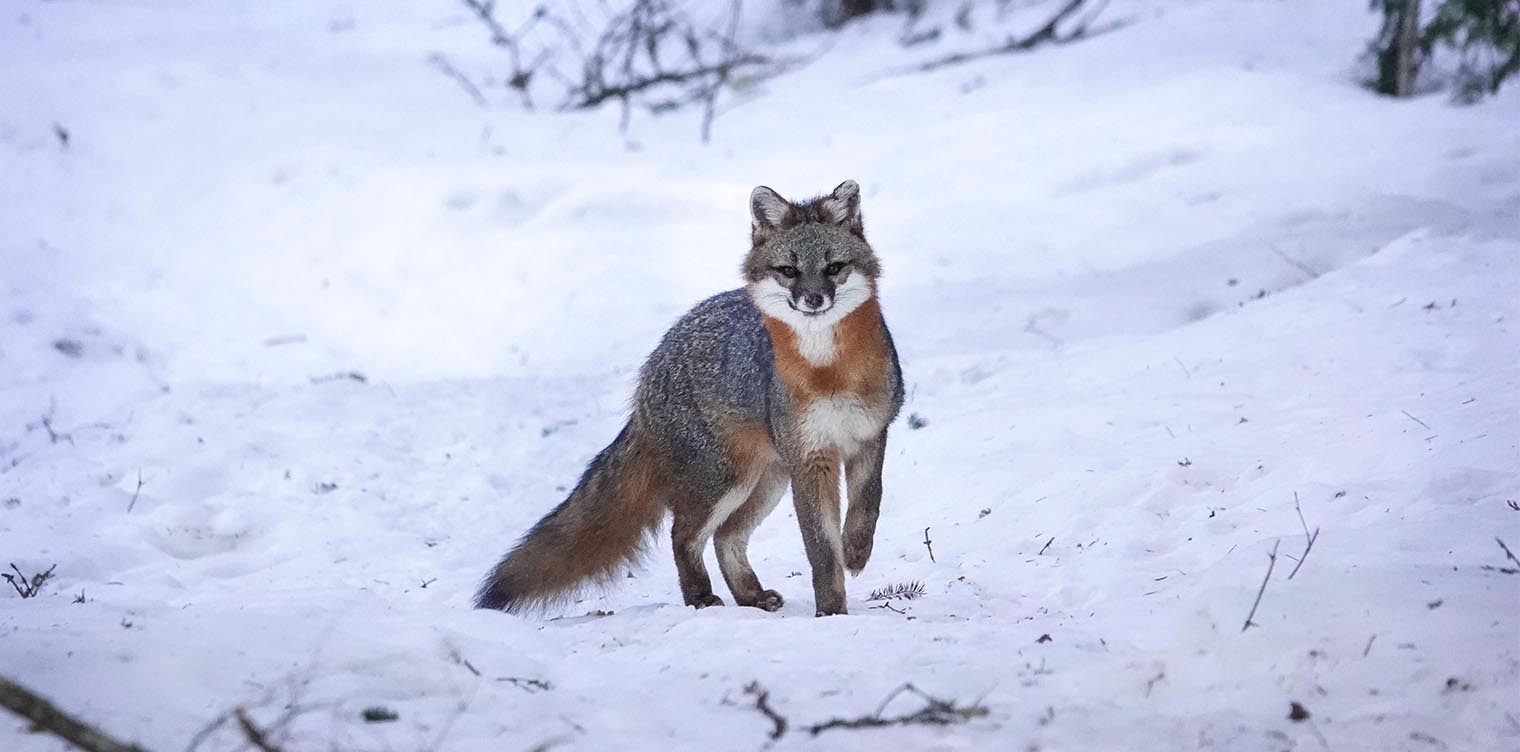The photograph captures a solitary fox standing in a snow-covered landscape. The fox is strikingly detailed with its distinct fur pattern: its back and the top of its head are primarily gray with various black spots, while its tail features a black tip and a mix of gray and dark orange fur. The underside of the tail and the front of its neck also exhibit vibrant orange tones. Its chest and stomach showcase large white spots, which also extend to its legs and under its mouth. The fox is positioned with its body angled to the right, but its head is turned towards the camera, giving it a direct, engaged look. One of its front paws is lifted, adding a dynamic element to its stance. The surrounding environment is a snowy terrain marked by various paw prints and patches of disturbed snow. Scattered bare branches protrude from the ground, and in the top right corner of the image, a tree is visible, still adorned with green leaves, contrasting against the otherwise wintry scene.